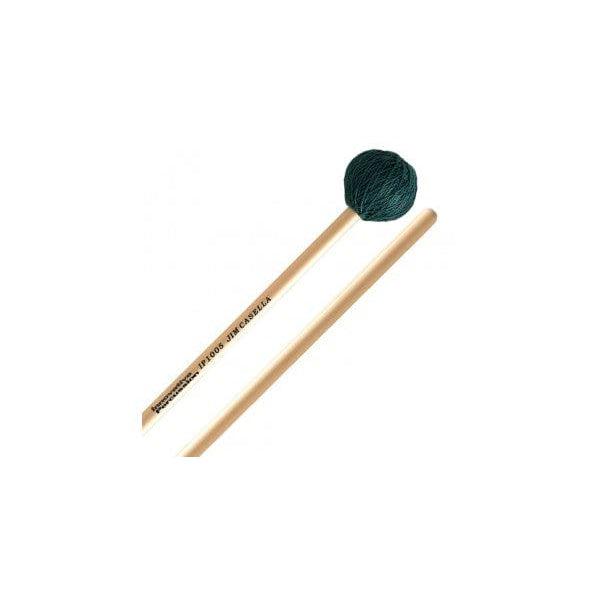The image depicts two light brown, thin wooden sticks against a plain white background. One of the sticks has a round ball of dark green yarn or thread affixed to one end, while the other end appears pointed. This stick also contains black text that reads "IP 1005 Jim Koscella" in capital letters, accompanied by some smaller, indistinguishable text. The second stick, which also has a pointed end, appears to lack any attached yarn or visible text. The overall colors in the image include tan, white, and dark green. The function of these sticks is unclear, though they resemble tools that could hypothetically be used for knitting or cleaning, although their exact purpose is uncertain.